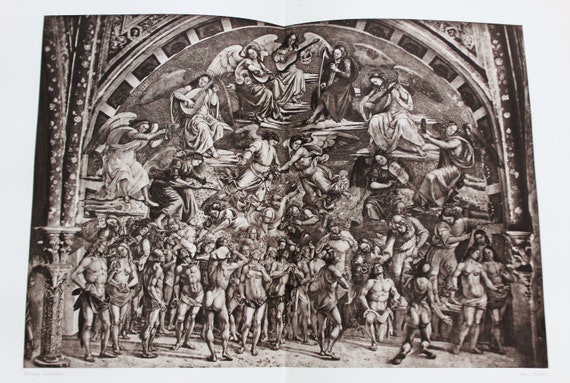The image is a monochromatic mural or drawing in shades of black, white, and grayscale, resembling a stencil or fresco style. It unfolds like an open book with a slight crease down the center against a grayish or off-white background. The artwork depicts a scene possibly evoking ancient or religious themes inside an arch-shaped or domed area. 

At the bottom, a multitude of muscular, unclothed men and a woman partially draped in small fabrics or toga-like cloths are gathered, some standing, some kneeling, with varied orientations—some facing forward, others with their backs turned, and a few facing the wall. 

Above them, a tier of angels in robes is seen, some seated on rocks and playing musical instruments. These angels appear to be looking down upon the crowd below, contributing to the celestial aura of the upper section. The intricate composition captures a profound contrast between the earthly figures at the bottom and ethereal beings above, all rendered in detailed black-and-white intricacy.